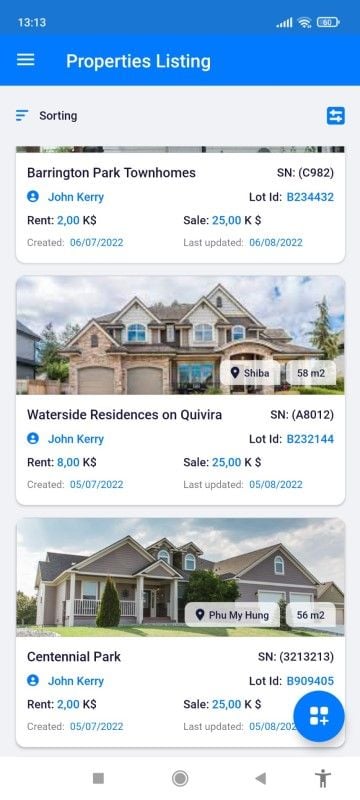**Detailed Caption:**

The image appears to be a screenshot taken from a mobile phone displaying a real estate listing app. At the very top of the screen, a blue status bar shows essential phone information, including the current time (13:13), signal strength, Wi-Fi connection status, and battery charge level, indicating that the device is charging. Just below this bar, there's a white header containing navigational elements; prominently displayed is the word "Sorting," which likely allows users to sort property listings based on various criteria. Next to "Sorting," there are three horizontal lines, suggesting additional options for sorting properties.

The main section of the screenshot features three separate property listings. Unfortunately, the very top listing is only partially visible, revealing just the property name, "Barrington Park Townhomes," realtor's name, "John Kerry," rental price of $2,000 per month, and purchasing price of $25,000K. This listing also includes an identifying lot ID number and timestamps indicating when the listing was created and last updated.

The second listing is fully visible, showcasing a property named "Waterside Residence on Quivira," which is a single-family home. John Kerry is once again listed as the real estate agent. The screenshot provides a sale price of $800K and mentions a rental option for $25,000K, though it seems there's some confusion with the rental terms. This listing also includes a lot ID number along with its creation date of May 7th, 2022, and last update on May 8th, 2022.

The third and final listing on display is for a single-family home in "Centennial Park," with John Kerry as the realtor. This property has a rental price of $200K and a purchase price of $25,000K. Like the other listings, this entry also gives its lot ID number along with the creation date of May 7th, 2022, and a last update date of May 8th, 2022.

At the bottom of the screenshot, there are several icons, one of which appears to be a back button, though the functionality of the other icons is not clearly identified in the description.